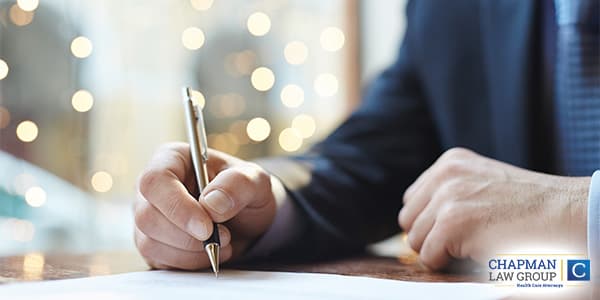This is a rectangular advertisement for Chapman Law Group. The image captures a man, shown from the shoulders down, seated at a wooden desk. He is intently writing on a piece of paper using a sophisticated metal pen, which features a gold top and a black grip. His right hand is balled into a fist, resting at the bottom of the paper. The man is dressed in a blue suit paired with a light blue checkered tie, and his white shirt cuffs are visible at the edge of his jacket sleeves. The background is deliberately out of focus, showcasing strings of circular lights that add a subtle ambiance to the scene. In the bottom right corner of the image, there is a watermark with a logo, presumably for Chapman Law Group, along with additional text that is too small to read. The emphasis of the composition is on the act of writing and the professional attire, underscoring the advertisement's legal theme.